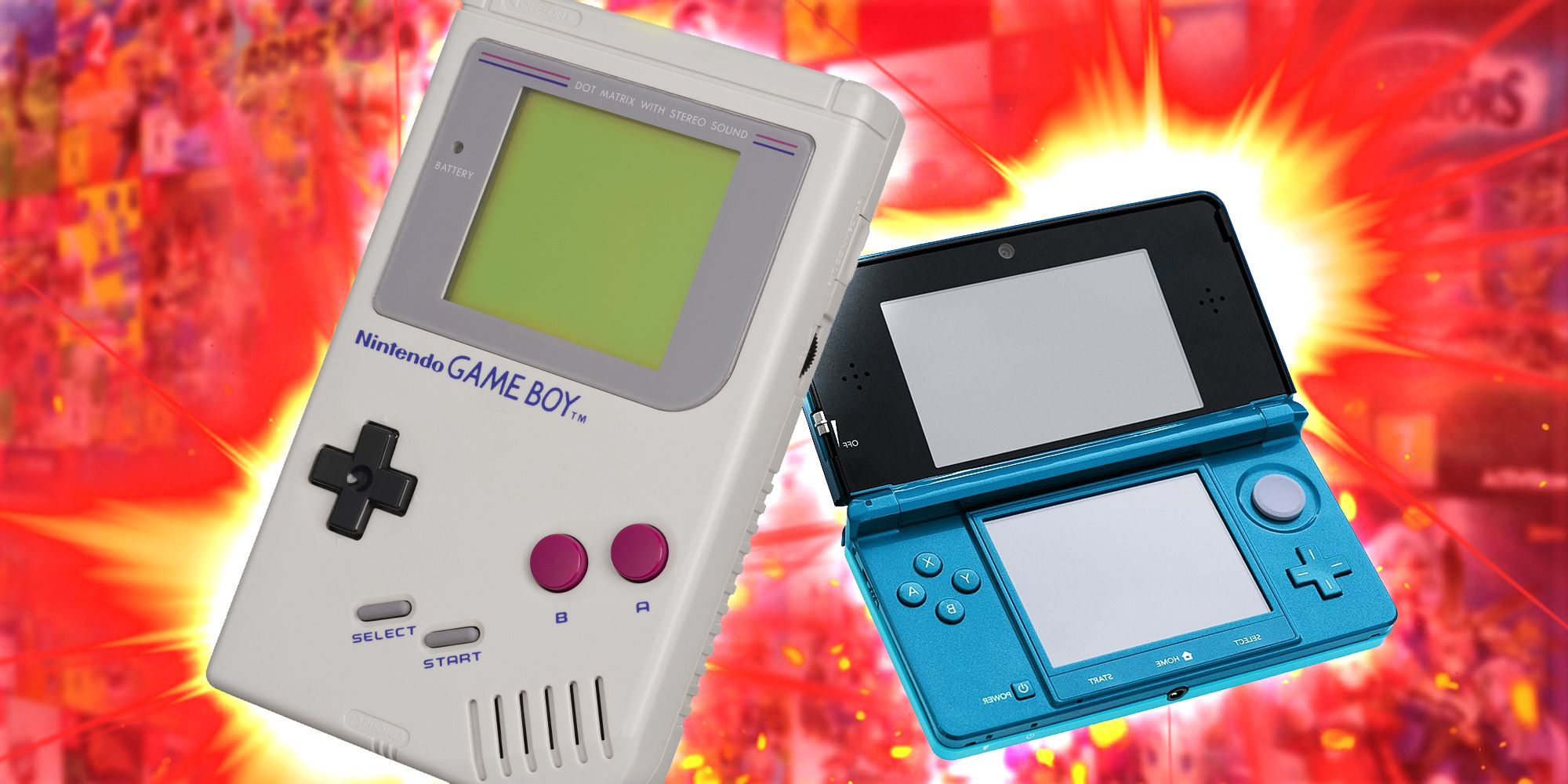In this vibrant image, two classic Nintendo handheld gaming devices are displayed against a striking background of abstract red and yellow explosion graphics, creating a dynamic "wow" effect. On the left, the original gray Game Boy, featuring a familiar black directional pad, two distinct red 'A' and 'B' buttons, and gray 'Select' and 'Start' buttons, displays its iconic green screen with a gray border and the label "Dot Matrix with Stereo Sound." On the right, partially covered by the Game Boy, sits a blue and black Nintendo 3DS. It boasts a modern dual-screen setup, complete with a circular directional stick, a traditional D-pad, and four action buttons labeled 'A,' 'B,' 'X,' and 'Y,' hinting at its advanced touchscreen technology and interactive capabilities. The vibrant red and yellow explosion graphic behind the devices adds an energetic backdrop, emphasizing the evolution of handheld gaming.